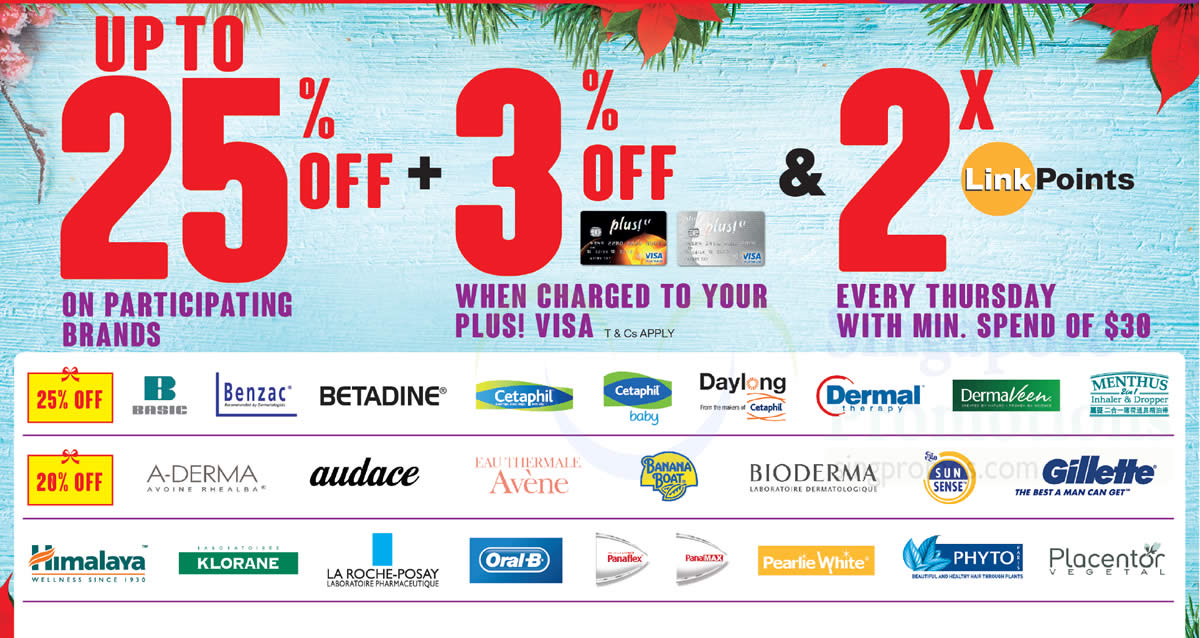**Detailed Sale Ad Description:**

The sale advertisement screen features a visually appealing background of light blue painted wood, with a noticeable texture emphasizing its rustic charm. Accentuating the backdrop are delicate red flowers paired with green evergreen pine tree boughs, artistically placed at the upper corners and center of the screen.

Prominently displayed in bold red text stretching from left to right, the ad highlights "Up to 25% Off" as the main offer. Just below this, in a contrasting shade of purple, the text reads, "on participating brands," indicating the scope of the promotion.

To the right, a black plus symbol precedes additional red text stating "3% Off." Beneath this, the ad informs viewers in purple text that the additional discount applies "when charged to your Plus Visa." Adjacent to this text, two stylized Plus Visa credit cards are depicted—one in a striking black and orange design, the other in a sleek silver and gray. Following these card images is a symbolic black ampersand and a red "2x," denoting a further promotional offer.

In purple text below this, the ad details, "every Thursday with a minimum spend of $30," specifying the conditions for the Thursday promotion. Nearby, a vibrant yellow circle with white text inside spells out "link," leading into black text that reads "points."

At the bottom of the screen, on a clean white background from left to right, various promotional details are laid out in yellow boxes:

- The first yellow box with red text announces "25% Off," listing participating brands: Basic, Benzac, Betadine, Cetaphil, Cetaphil Baby, Daylong Cetaphil, Dermal Therapy, Dermavine, Memphis Inhaler and Dropper.
- Following this, another yellow box with red text indicates "20% Off" for brands such as Aderma, Odachi, Euthermal Avane, Banana Boat, Bioderma, Sunsense, and Gillette (notably including their tagline, "the best a man can get").
- Beneath this, the discount applies to brands like Himalaya, Chlorane, La Roche-Posay, Oral-B, and Panaflex. The offer concludes with Panamax, Pearly White, Phyto, and Placentor Vegetal.

This detailed and structured layout ensures clear visibility and understanding of the diverse promotional offers available.